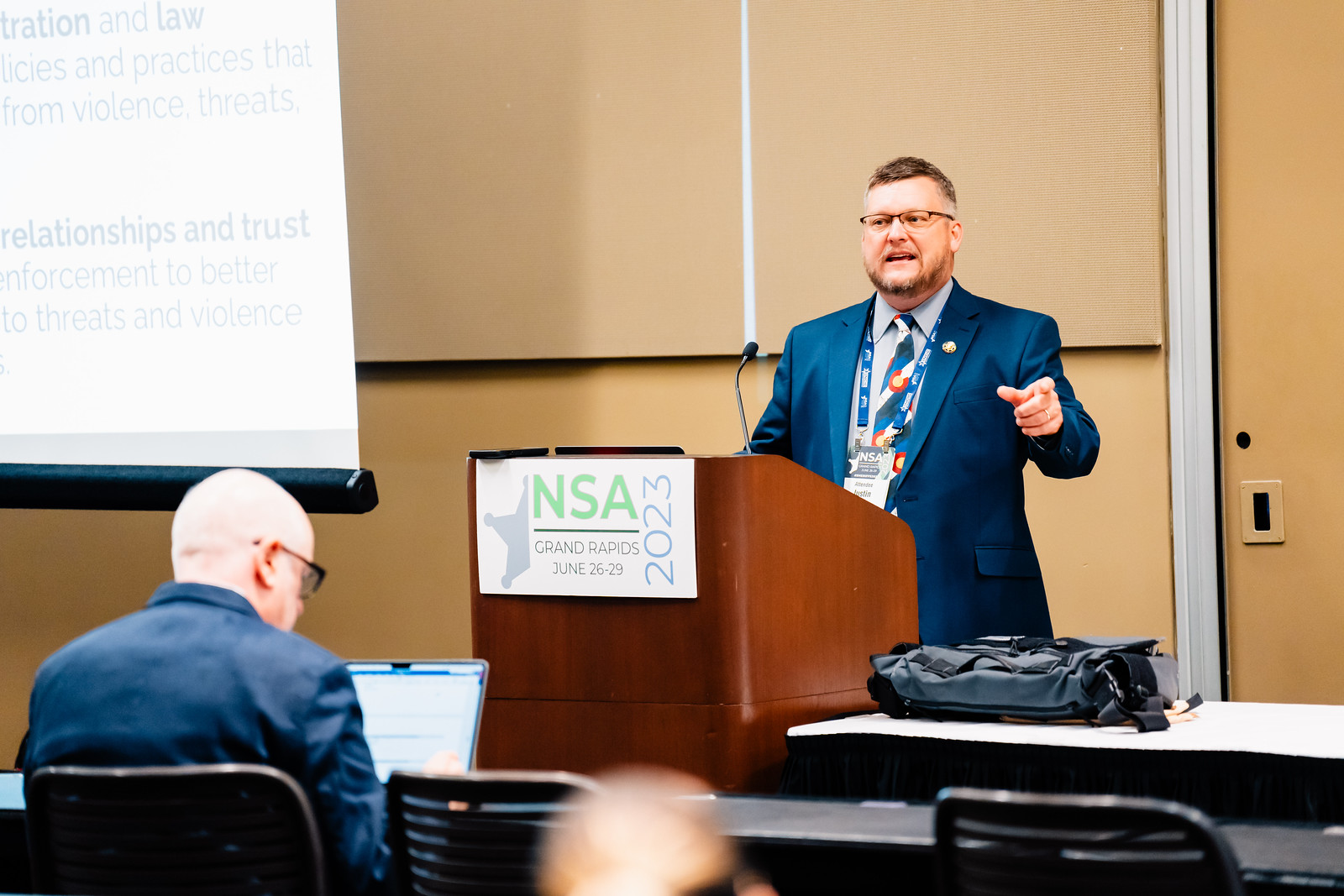This horizontally aligned, rectangular color photograph captures a business meeting or conference taking place indoors in a conference room. Dominating the right side of the image, a mid-aged white male speaker, possibly in his late forties or early fifties, stands behind a brown wooden podium, gesturing with his left hand, indicative of an impassioned speech. He sports a neat beard, short hair, wire-rimmed glasses, and is dressed in a navy blue blazer, a lighter blue collared shirt, and a blue and white plaid tie. Around his neck hangs a blue and white lanyard. Attached to the front of the podium is a sign with green capital letters "NSA," a blue "2023" along the right side, a partial blue star on the left, and below that, smaller black text reading "Grand Rapids" and partially legible dates in June.

To the left of the speaker, a white projection screen hangs on the upper left side of the wall, displaying partially readable phrases like "relationships and trust," "law," "seize and practice," and "threat and violence." Beneath and in front of the projector screen sits another white male, likely in his early fifties with a short haircut or bald head, wearing a black blazer and spectacles. He faces a flat laptop screen and sits in a dark office chair, flanked by additional horizontal-slatted chairs. 

The background features a tan-paneled wall and a locked door. In the foreground, rows of tables and chairs face the speaker, with two men visible. One is a Caucasian male with a bald head, out of focus at the bottom center, and the other, an older gentleman with glasses and a blue blazer, appearing engrossed in the presentation. This detailed image typifies a professional business environment in the United States in 2023, emphasizing the serious and focused nature of the ongoing discussion.